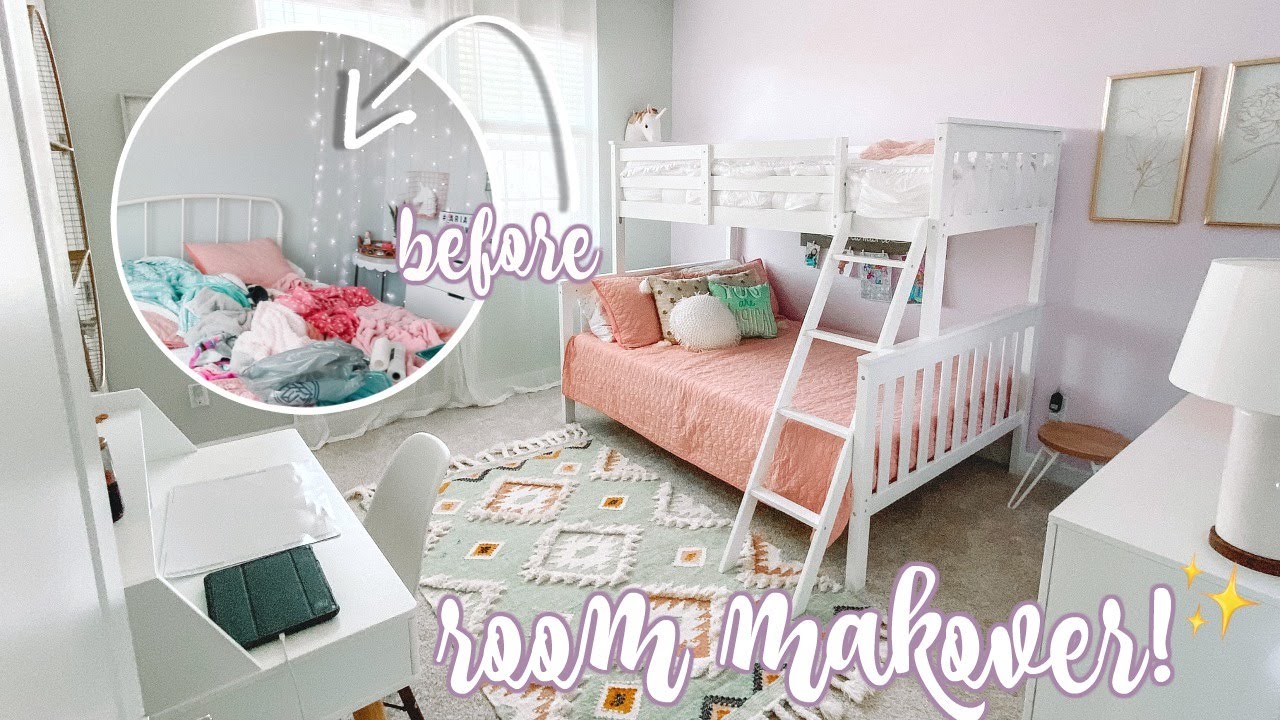This is a detailed photo for a room makeover, likely intended for internet platforms like Instagram or possibly a magazine or website. It features a transformational "before and after" layout. The larger "after" photo depicts a clean and organized room, possibly a guest room or a young adult's room, designed with a soft and airy aesthetic. The walls are painted a pale pink, adding a touch of warmth.

A white wooden bunk bed dominates the room, with a peach-colored bedspread adorned with coordinating pillows in shades of white, green, and pink. The top bunk, accessible via a white ladder with rungs at the foot, has white bedding complemented by a pink sheet and a stuffed animal. 

To the left of the bunk bed sits a pristine white desk paired with a matching white chair, setting a neat workspace vibe. On the floor, there’s a woven rug with diamond patterns that adds texture to the space. To the right, a white dresser topped with a white lamp rounds out the furniture. The room also features two pieces of art hanging on the wall, enhancing its aesthetic appeal.

The inset "before" photo, marked by a white circular frame and labeled "before" in a cursive calligraphy style with a sparkling emoji, depicts a chaotic scene. It shows a bed piled high with clothes and miscellaneous items, sharply contrasting the tidy "after" photo. 

Overall, the makeover transforms the room into a serene and orderly space, with a cohesive color scheme of white, peach, and green, seamlessly blending functionality and style.